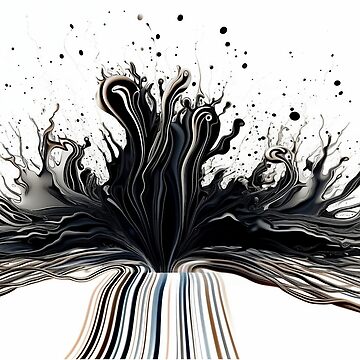The image is a digital painting showcasing an abstract design. Set against a pure white background, the lower third of the artwork is occupied by an array of vertical, slightly wavy lines of various colors and thicknesses. These lines include shades such as light brown, black, dark blue, light blue, tan, yellowish, and pinkish hues. The lines converge into a dynamic black splotch or splash located centrally but extending upward, resembling an ink explosion. The black splotch features jagged, splash-like edges and seems to burst out in multiple directions. Black circles and droplets of varying sizes emanate from this central splash, forming an arc across the top part of the image, mimicking the unpredictable scattering of ink droplets. The overall composition gives an impression of an ink eruption, with the lines leading up to the central explosion creating a dramatic visual effect, emphasizing the abstract nature of the artwork.